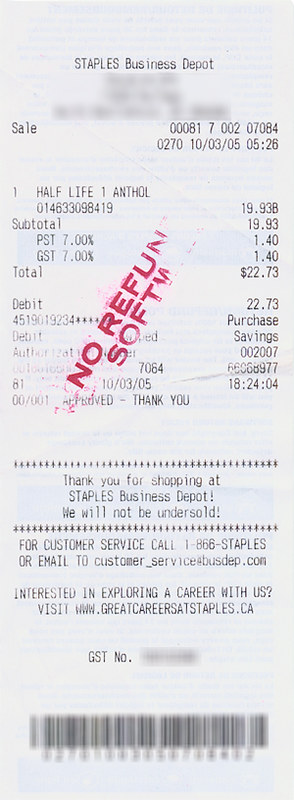The image features a vertically aligned, rectangular receipt from Staples Business Depot. The white receipt, imprinted with black text, lists the store name at the top, followed by the date, October 3rd, 2015, and the time, 5:26 PM. The main transaction details indicate the purchase of "Half Life 1 Anthol," likely a video game anthology, amounting to $19.93. Additional charges include a Provincial Sales Tax of $1.40, bringing the total to $22.73. A prominent red stamp at about a 70-degree angle reads "No Refund" and partially obscures the word "Software," identified by the visible letters "S-O-F-T." The payment was made using a debit card, partially redacted as 4519019234 followed by asterisks. The receipt concludes with a message of appreciation: "Thank you for shopping at Staples Business Depot. We will not be undersold." Customer service details include a phone number (1-866-STAPLE) and a website for career opportunities (www.greatcareersatstaple.ca), above a barcode located at the bottom.